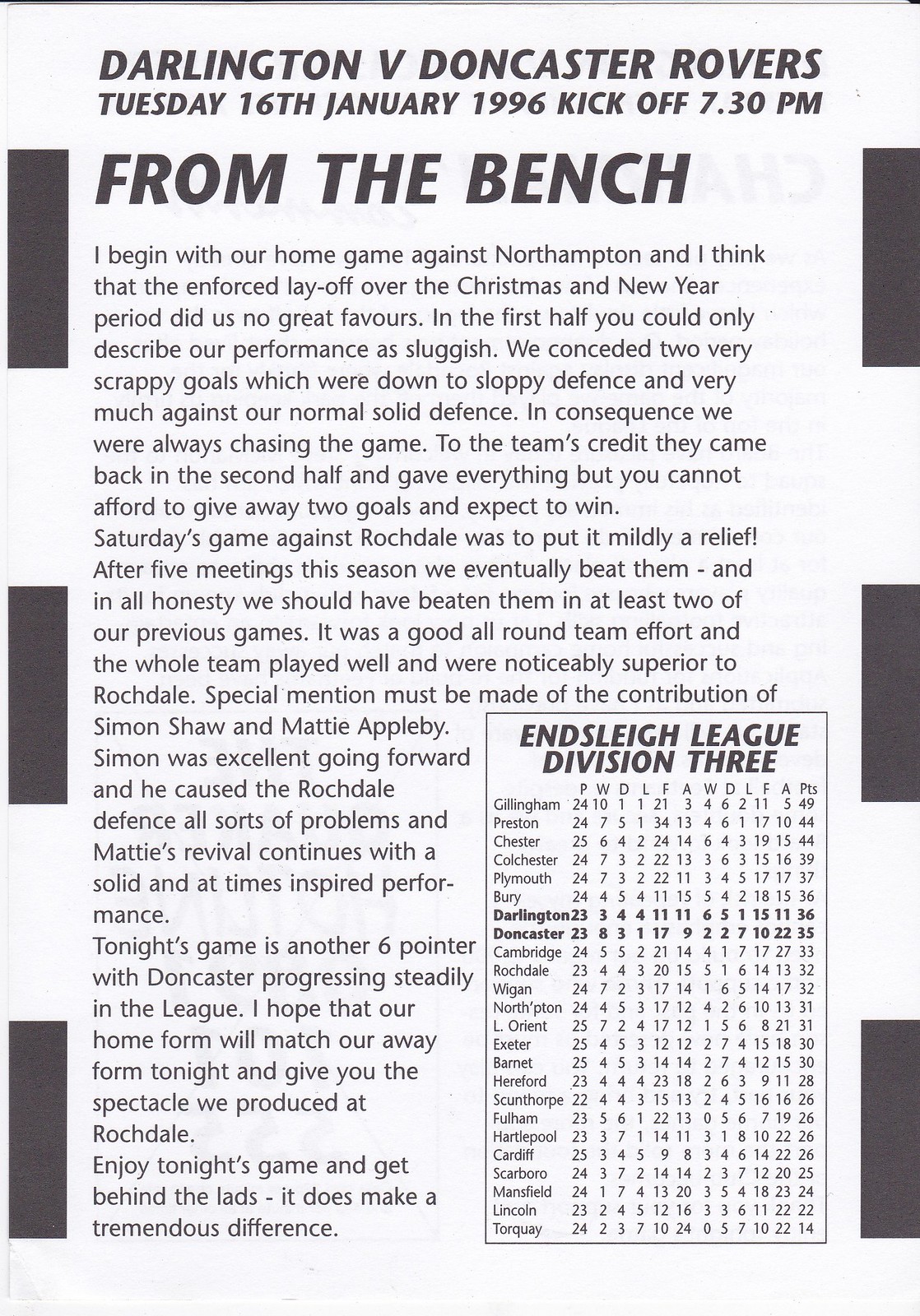This page from a British soccer program or magazine, presented in a black-and-white scan, showcases a detailed overview of a past match between Darlington and Doncaster Rovers held on Tuesday, January 16th, 1996, with a kickoff time of 7:30 p.m. The page features a white background with a distinctive black-and-white rectangular border on the left and right edges. At the top, the title "Darlington v. Doncaster Rovers Tuesday 16th January 1996 kickoff 7:30 p.m." is prominently displayed. Beneath it, in large, bold, capital letters, it reads "FROM THE BENCH."

The article starts with a reflection on a home game against Northampton, noting the adverse effects of a forced break over the Christmas and New Year period, leading to a sluggish first-half performance. The author mentions conceding two scrappy goals due to sloppy defense, a stark contrast to their usual solid backline. However, the team's commendable effort to fight back in the second half is highlighted, though ultimately insufficient to overcome the two-goal deficit.

Further detailed within the lengthy article is a recap of a game against Rochdale, where after several meetings, the team finally secured a victory. There's praise for the overall team performance, particularly highlighting the contributions of Simon Shaw and Mattie Appleby, the latter noted for a solid and occasionally inspired display. The piece concludes with anticipation for the match against Doncaster, expressing a hope that the team's current home form would mirror their successful away form.

In the bottom right corner of the page, there is a chart titled "Endsleigh League Division III" containing various statistics and last names likely belonging to teams or players, with "Darlington" and "Doncaster" emphasized in bold. The structured layout and detailed narrative encapsulate a moment in British football history, providing a robust context for the matches and player performances leading up to the highlighted game.